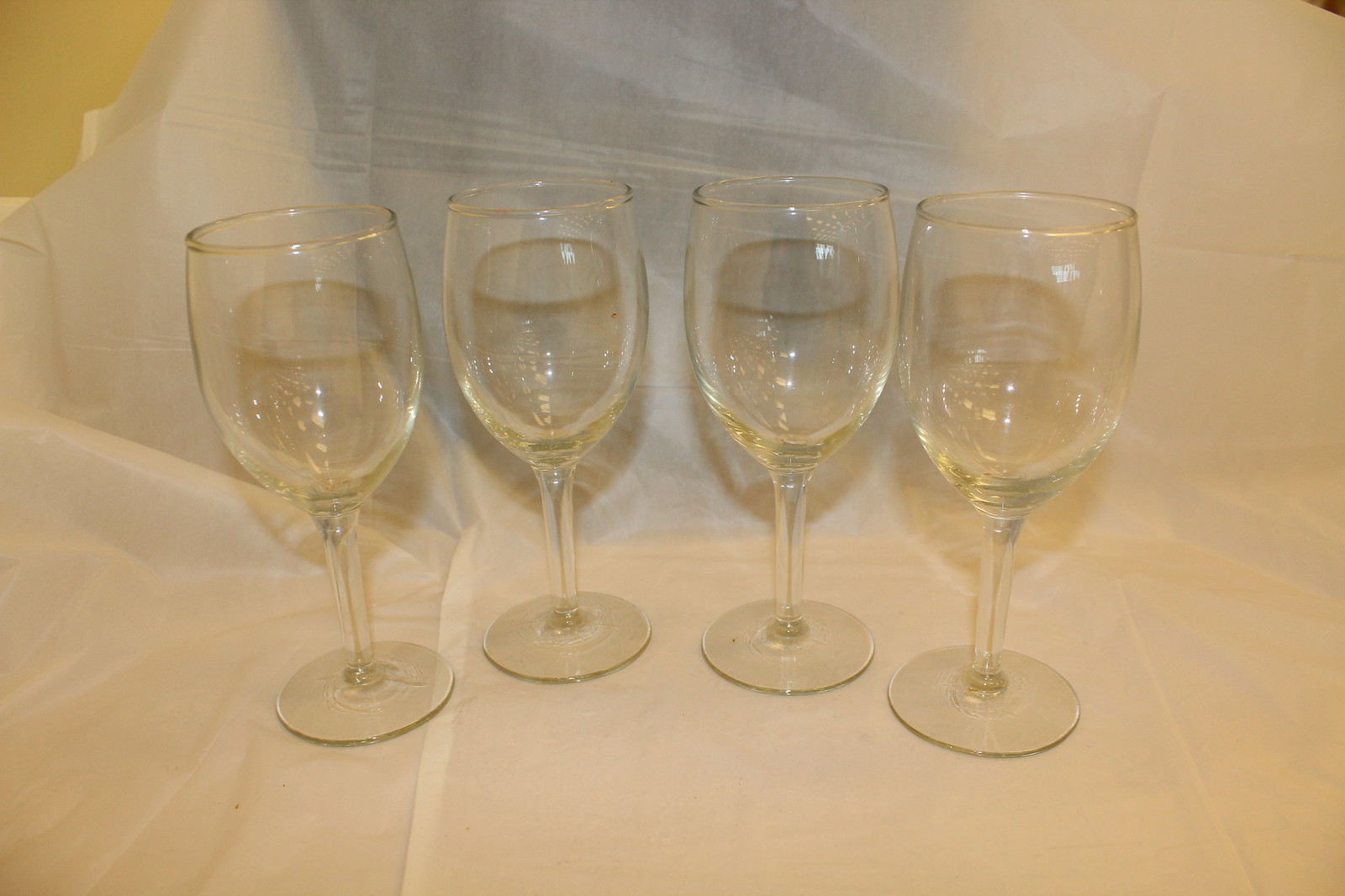The photograph features four matching, medium-stemmed wine glasses arranged in a row from left to right. Each glass has a gold-edged rim, and appears to be empty, without any wine or water inside. The glasses are placed on a piece of fabric that seems to be draped over a dark object beneath it, resembling a makeshift backdrop. The fabric features a pastel pattern that might evoke the look of a shower curtain or a decorative tablecloth. The backdrop is a plain white paper, but in the upper left corner, a yellow wall peeks through. The glasses themselves have a slight yellow tinge and may even have some brownish stains or shadows within them, suggesting they are of average quality. This image could be a creatively staged photograph for a personal or commercial purpose, such as listing the glasses for sale on an online marketplace like eBay.